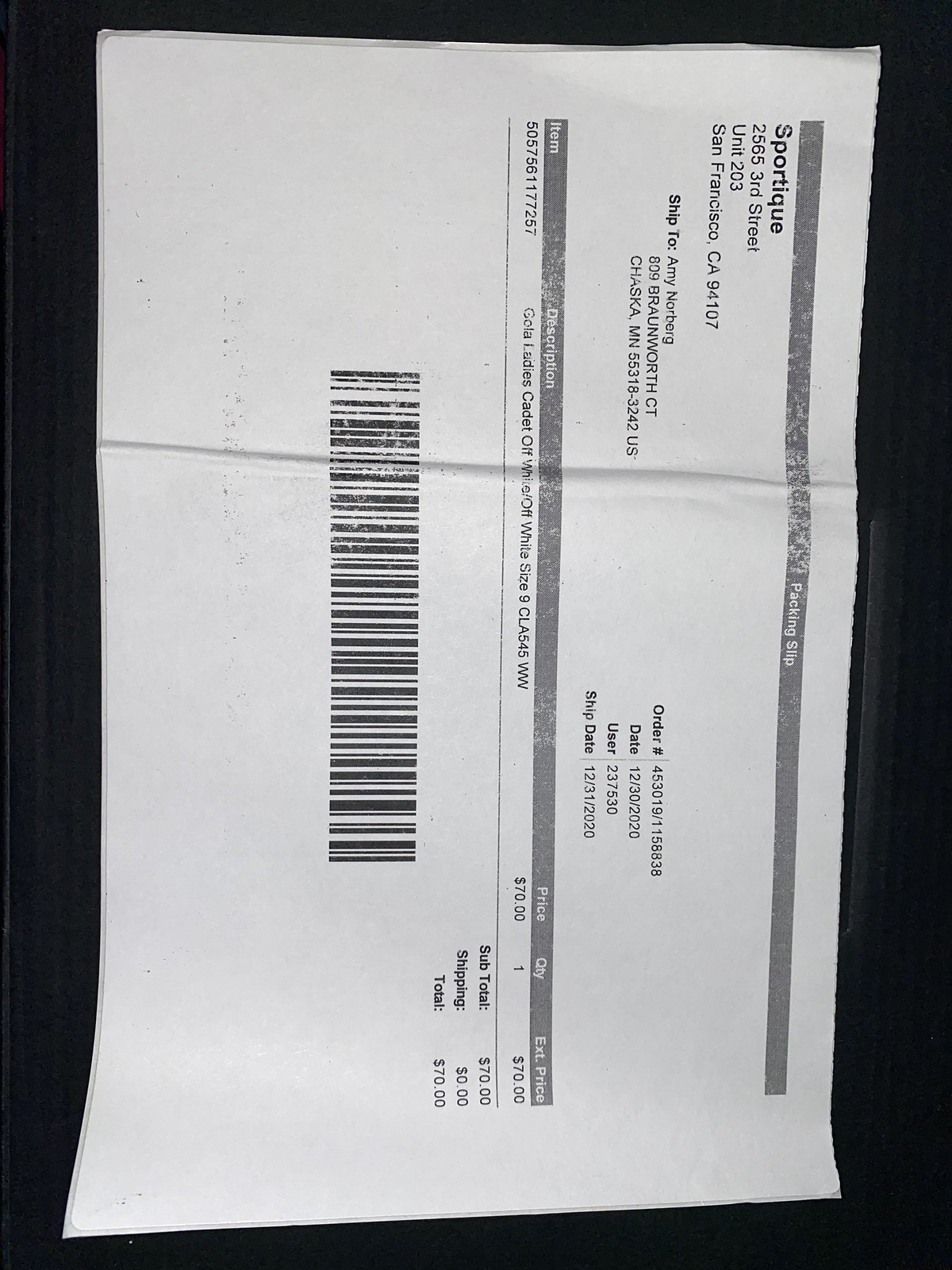A photograph of a packing slip printed on a half sheet of sticker label paper. The top of the slip indicates it originated from Sportique. Detailed transaction information is provided, confirming the purchase of GOLA Ladies Cadet sneakers in Off-White, size 9, model number CLA 545WW, priced at $70. The total cost of the order was $70, as shipping was free. The order was placed on December 30, 2020, and it was shipped on December 31, 2020. A barcode is prominently displayed at the bottom of the slip.